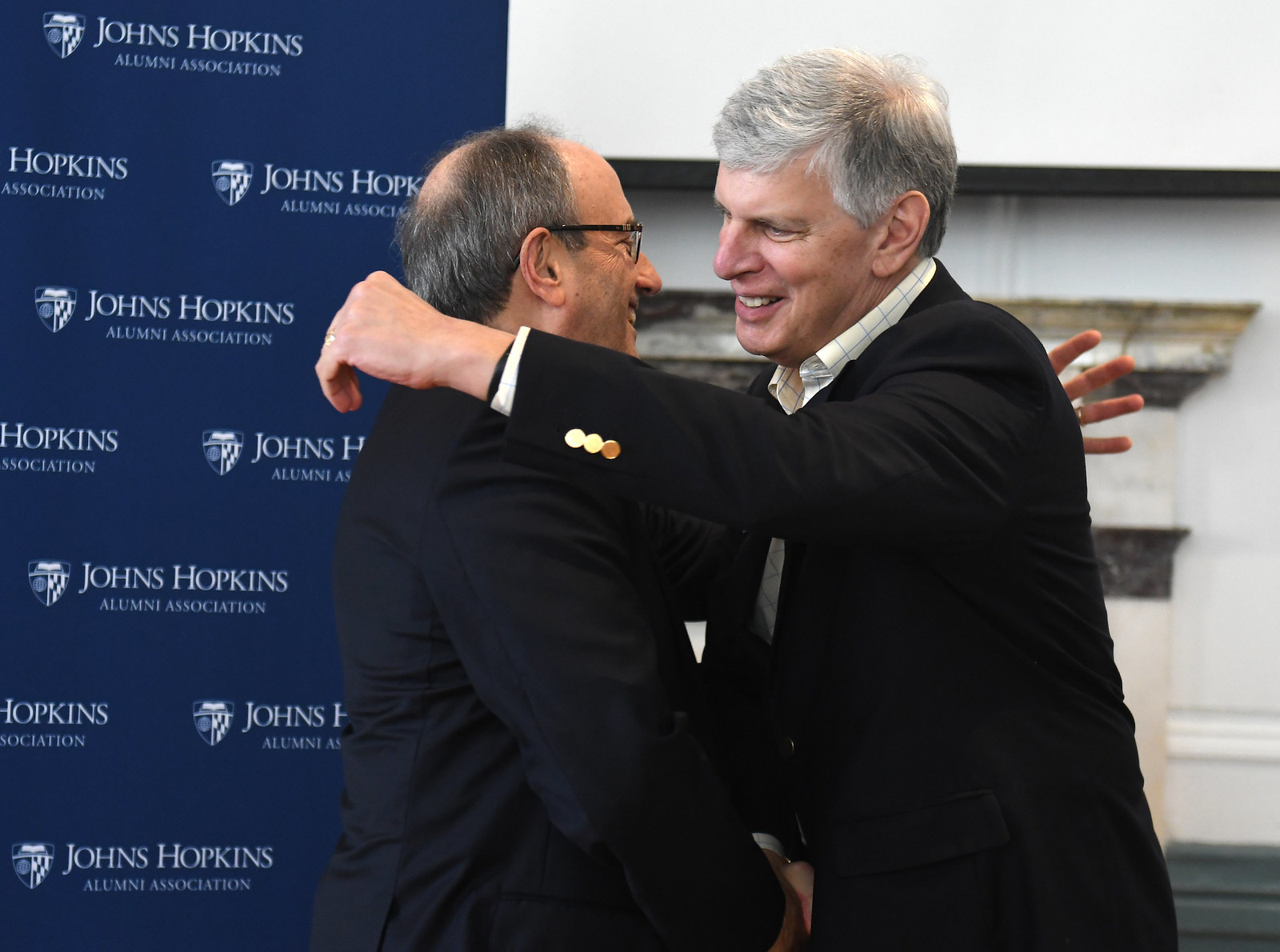In the photograph, two older men, both appearing to be in their fifties, are warmly embracing and shaking hands, suggesting a reunion or heartfelt greeting. Both are dressed in formal black suits; the man on the left is distinguished by his dark-framed glasses and balding head, while the man on the right has grayish hair and is adorned with gold cufflinks and a white undershirt. Their interaction is friendly and intimate, with one arm over each other's shoulders. 

The backdrop features a navy blue banner prominently displaying the words "Johns Hopkins Alumni Association" in white text. The text "Johns Hopkins" is in a larger font, with "Alumni Association" centered beneath it. Additionally, the banner includes the repeated crest or shield of Johns Hopkins University. The banner occupies the left third of the image, while the rest of the background includes a wall with white and black shelving. The overall setting indicates an alumni event for Johns Hopkins University.